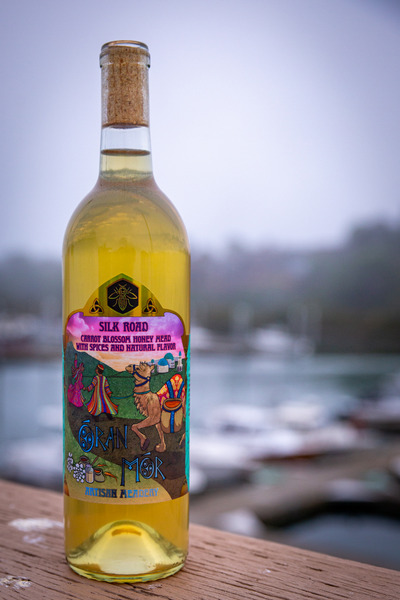In this daytime outdoor image, a clear glass bottle filled with a golden yellow beverage takes center stage in the foreground. The bottle is positioned on the left-hand side of a light brown wooden table or railing, tilted slightly at about a 30-degree angle from right up to the left. A long wooden cork tops the bottle, which features a prominent label. The label, shield-shaped at the top and rectangular in the center, reads "Silk Road, Carrot Blossom Honey Mead with Spices and Natural Flavor, Artisan Meadery." A picture of a camel with what looks like two men pulling it adorns the label. The background of the image is out of focus but hints at a picturesque scene of a body of water, white sailboats moored to a dock, and a distant tree line, all blurred to direct attention to the bottle. The colors in the image include the bottle's golden yellow contents, the light brown of the wooden table, and an array of soft hues, including off-white, blue, violet, and orange, subtly indicating a tranquil outdoor setting.